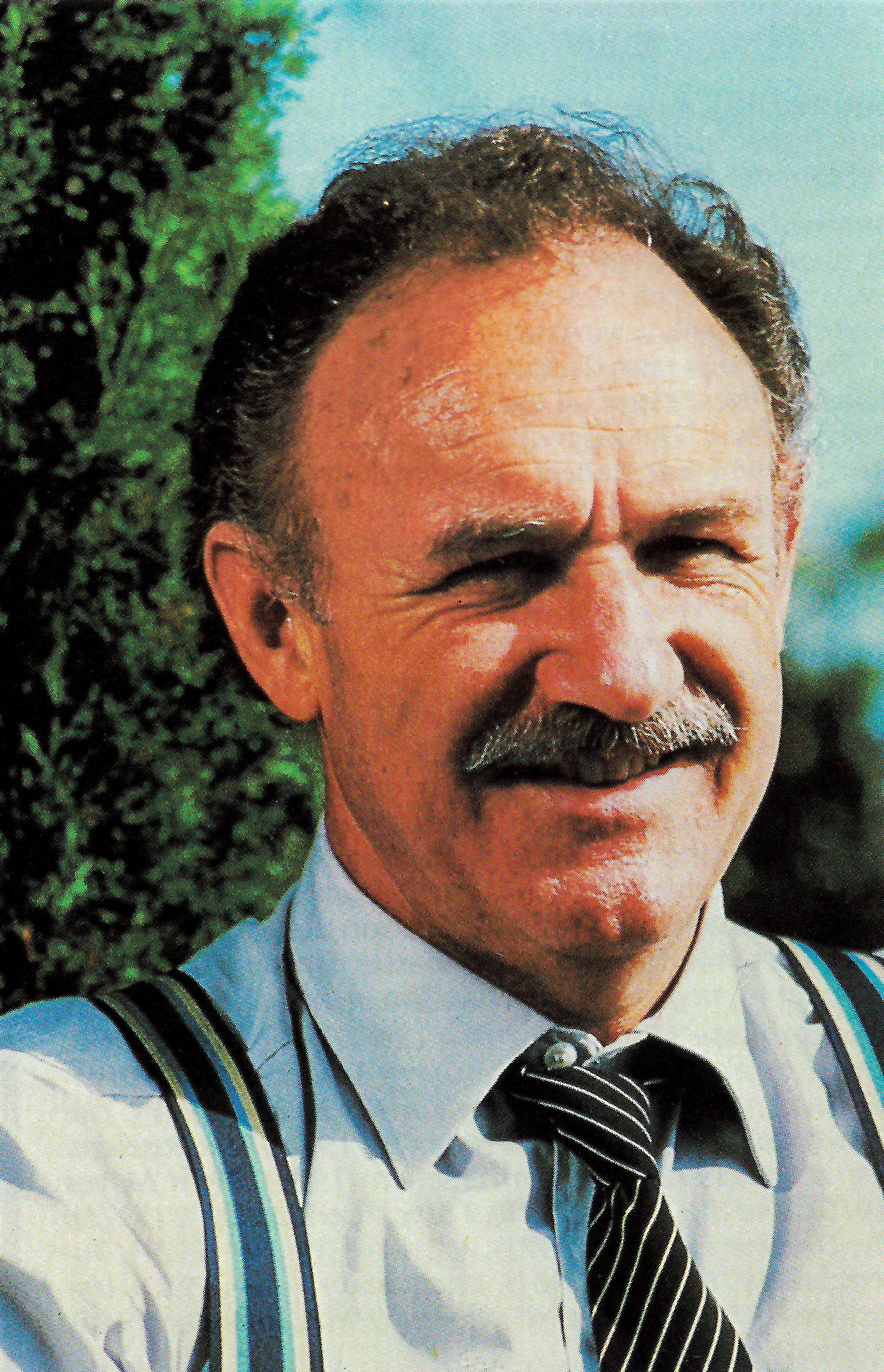The image depicts a vintage photograph of a distinguished older, white man, most likely a well-known actor who closely resembles Gene Hackman. The man sports a salt-and-pepper mustache and is balding with a mix of brown and gray hair. He is wearing a light blue, collared button-down shirt with the top button undone, paired with navy blue, striped suspenders. A black tie adorned with white stripes completes his attire. The man is squinting slightly, possibly due to the sun, and smiling gently at the camera, adding a touch of warmth to his expression. Behind him, there is a green shrub or small tree, with a bright blue sky visible above, indicating that the photograph was taken outdoors on a sunny day. Wrinkles on his face hint at his age, contributing to the timeless quality of the photograph.